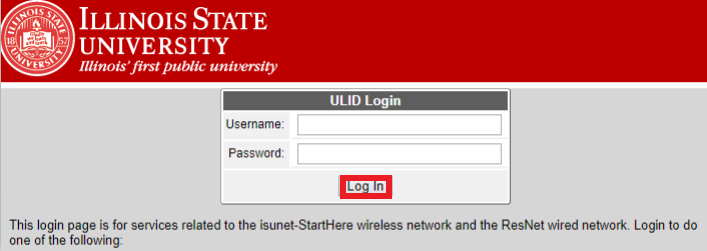The image showcases a login page for Illinois State University with prominent school branding and instructions. At the top, a red horizontal strip features the text "Illinois State University, Illinois' first public university" in bold white lettering. Adjacent to this text is the university’s circular emblem, which depicts an open book and includes the words "Illinois State University" in red, white, various shades of gray, and black.

Below the red strip, the background shifts to a neutral gray. Centered on this gray backdrop is a large, horizontally oriented rectangle box. Inside this box, instructions and input fields are displayed. At the top of the rectangle, "ULID Login Username" is written, followed by an empty user field. Beneath this is "Password," accompanied by another empty field for input. Both fields are devoid of any text.

A prominently outlined red button labeled "Login" anchors the bottom of the rectangle, catching the viewer’s eye.

Outside the rectangle, still on the gray background, there are additional instructions reading: "This login page is for services related to the isunet.starthere wireless network and the renet wired network. Login to do one of the following: ..." However, this text appears to be truncated, with part of the message cut off and not visible in the image.